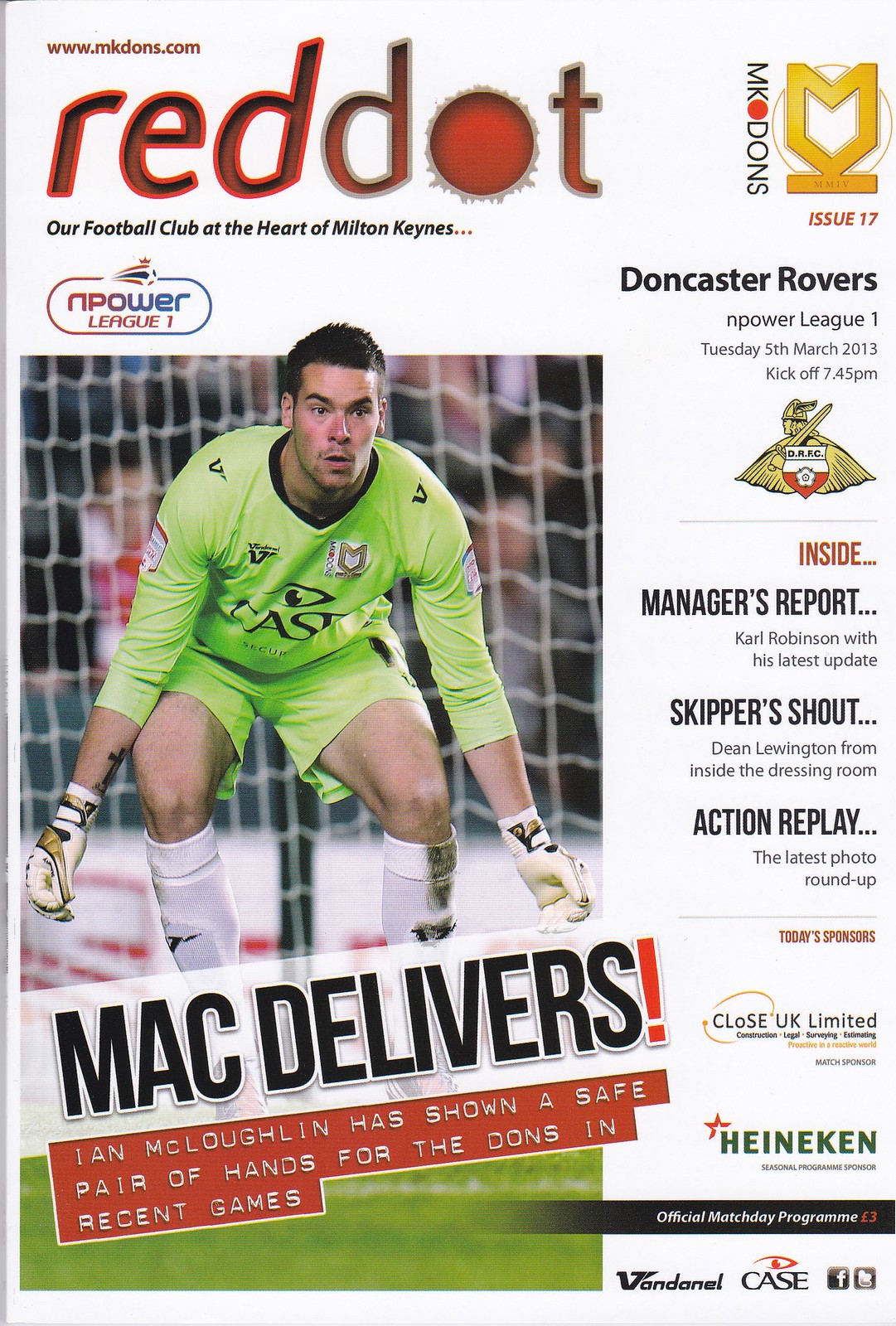The image shows the cover of a football (soccer) article publication against a white background, accented with vibrant colors. On the left-hand side, there is a dynamic action shot of a soccer goalie. The goalie, a Caucasian male, is depicted mid-jump in front of the goal. He is dressed in a light green shirt and shorts, complemented by white socks and gloves.

The accompanying text states, "MAC DELIVERS, IAN MCLACHLAN HAS SHOWN A SAFE PAIR OF HANDS FOR THE DONS IN RECENT GAMES," and is rendered in black and red fonts, with parts of it set against white and red backgrounds.

The name of the publication, "REDDOT," is prominently displayed at the top in a bold red and black font. Below this title, a subheading reads, "OUR FOOTBALL CLUB AT THE HEART OF MILTON KEYNES, N-POWER LEAGUE 1."

On the right-hand side of the cover, additional information is provided. It includes the issue details, "MCDONS ISSUE 17," the opposing team "DONCASTER ROVERS," the league "N-POWER LEAGUE 1," and the match date and time, "TUESDAY THE 5TH OF MARCH 2013, KICKOFF AT 7.45 PM."

Inside the publication, readers can expect:
- MANAGER'S REPORT featuring Carl Robinson's latest update.
- SKIPPER'S SHOUT with insights from Dean Lewissting inside the dressing room.
- ACTION REPLAY offering the latest photo roundup.
- TODAY'S SPONSORS, identifying Close UK Limited and Heineken.

At the bottom right corner, it indicates the publication is an "OFFICIAL MATCHDAY PROGRAM," priced at 3 Euros. Additionally, various brand logos are present, including those labeled "VAN DANEL" and "CASE," alongside Facebook and Twitter logos, suggesting social media presence.

Overall, the cover blends engaging visuals and informative text, capturing the essence of an exciting matchday experience.